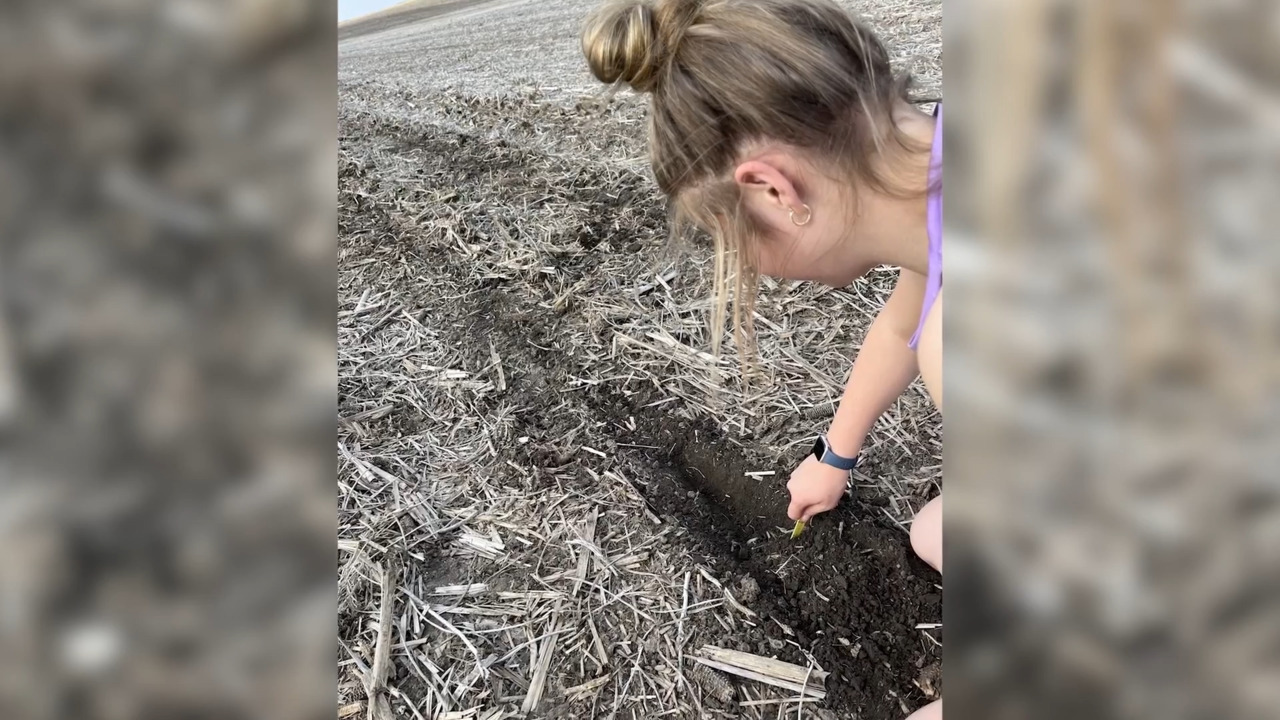The image depicts a close-up view of a woman, with a light skin complexion and brown and blonde hair pulled into a bun, working outdoors in a field of rich, dark brown soil covered with straw. The scene is bright and clear, indicating it is daytime. The woman, who is wearing a purple tank top, has a smartwatch on her right wrist and appears to be using a tool to dig into the soil, perhaps preparing the field for planting crops. The background shows tire tracks running through the straw, and the left and right borders of the image are blurred, giving an impression of depth and extending the field's appearance.